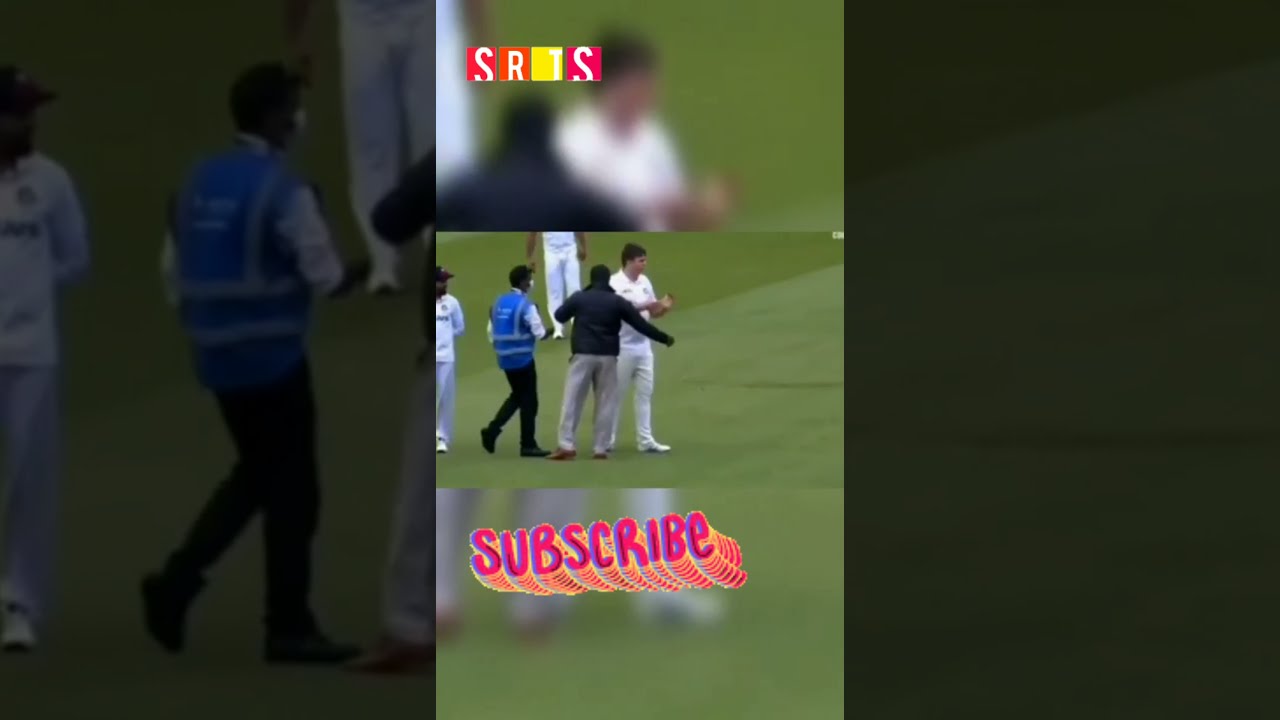The image depicts a scene from a grassy field, likely a sporting venue, featuring a small group of people. At the center of the image, a person in a black jacket and khaki pants faces a person dressed entirely in white, who is wearing a short-sleeved shirt and long white pants with matching white shoes. To the left of the individual in the black jacket stands a person in a royal blue safety vest, paired with black pants and black shoes, appearing to approach the black-jacketed individual. All figures are engaged in a conversation or discussion. Above the scene, there is text that reads "SRTS" in white letters on a yellow rectangular background, arranged in a ransom-letter style, while the bottom of the image contains the word "SUBSCRIBE" in hot pink letters set against a peach-colored background. The image itself is oriented in landscape format.